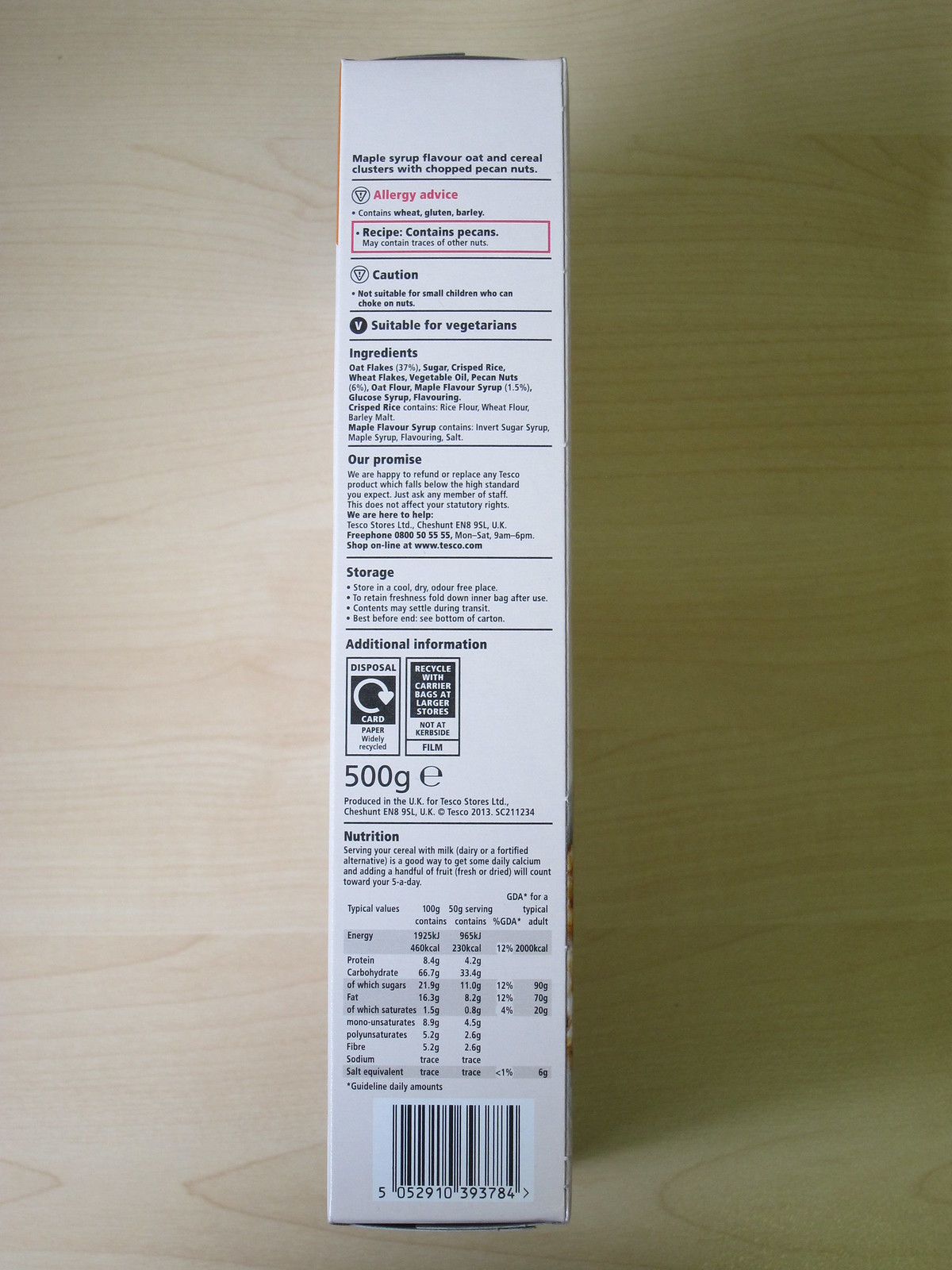The image captures the thin side of a large, white, cardboard box lying on a pale wooden surface, showcasing a detailed ingredient label and nutritional content for a granola-style snack. At the top of the box, "Maple Syrup Flavor Oat and Cereal Clusters with Chopped Pecan Nuts" is prominently displayed. This indicates a trail mix or granola bar enriched with pecans. Beneath this, in gray text, the heading "Allergy Advice" precedes a warning that the recipe contains pecans. Further down, in black text, it states the product is suitable for vegetarians.

The extensive ingredient list begins with oat flakes and sugar as primary components. Nutritional information reflects a caloric content of 200 calories per 100 grams, with the total product weighing 500 grams. A barcode is visible at the bottom of the box. Detailed sections delineating storage instructions, additional information, and disposal guidelines are mentioned, although the text is too small to be legible in the image. Overall, the box's design features black font on a white background, with "Allergy Advice" notably highlighted in red ink.